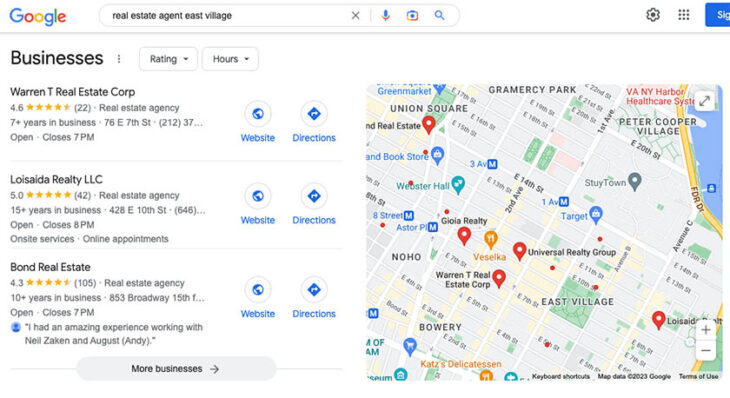A Google business search for "real estate agent East Village" is displayed at the top of the screen. The search bar and most of the page appear on a white background, although the image is cut off on the right side, preventing the full screen from being seen. The visible portion shows several business listings. 

On the left, three real estate agencies are prominently featured:
1. Warranty Real Estate Corp: 
   - 4.6 stars, based on 22 reviews
   - Described as a real estate agency with over seven years in business
   - Includes a visible website link and an option for directions
   - Operates until 7:00 PM
   
2. Louisa IDA Realty LLC:
   - 5 stars, with 42 reviews
   - Operating for over 15 years
   - Offers on-site services and online appointments
   - Closes at 8:00 PM

3. Bond Realty Estate:
   - 4.3 stars, based on 105 reviews
   - Listed as a real estate agency

On the right side of the screen, there is a map with pins marking the locations of five real estate agencies, although three additional results remain hidden. The map features a variety of pin colors including red, orange, blue, green, gray, and yellow.